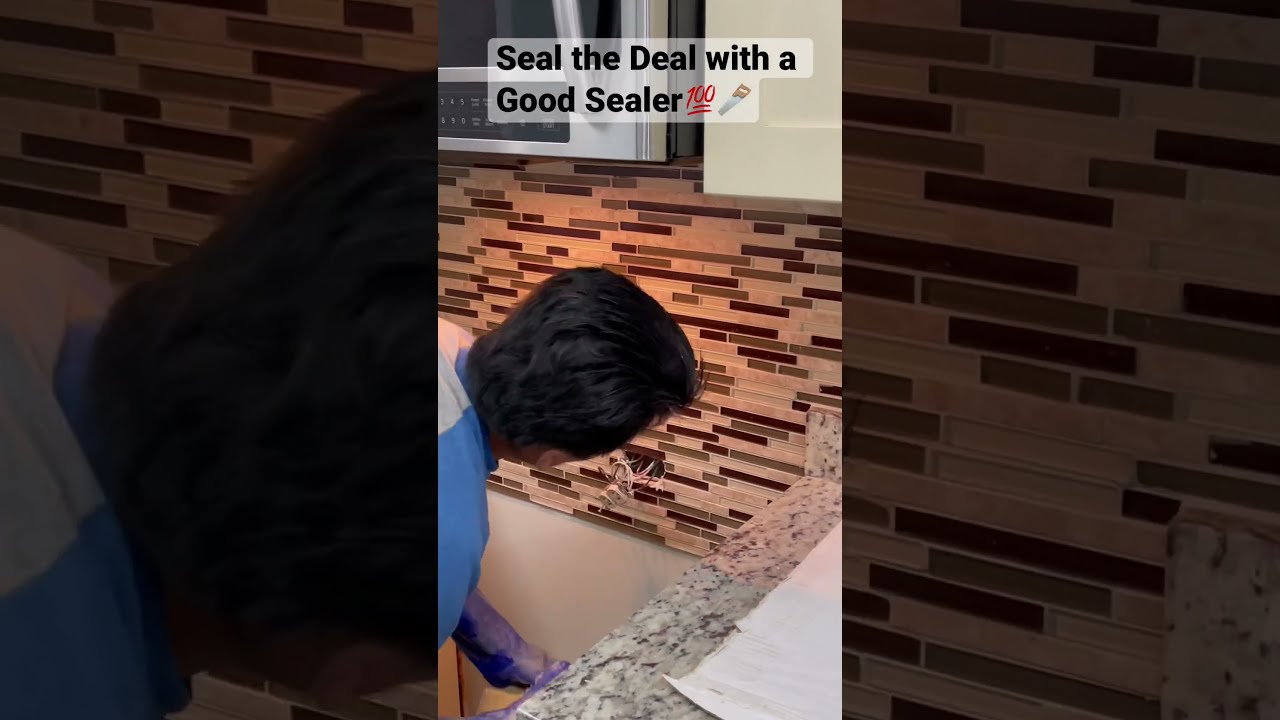The image is divided into three vertical sections, with the first and third sections displaying darkened close-ups of the central image. The central section features a photograph of an indoor scene, where a man with black hair, dressed in a white and blue t-shirt, is bent over, revealing the back of his head and shoulders. He appears to be working on an electrical outlet embedded in a tiled wall, from which a tangle of wires protrudes. A granite countertop is visible in the lower right portion of the image. Above the photo, superimposed text reads, "Seal the deal with a good sealant," accompanied by the "100" emoji underlined in red and a saw emoji. The backdrop of the text is white rectangles, and there appears to be a window in the setting. The tiles on the wall exhibit thin rectangles in various shades of red and brown, contributing to the overall indoor atmosphere.